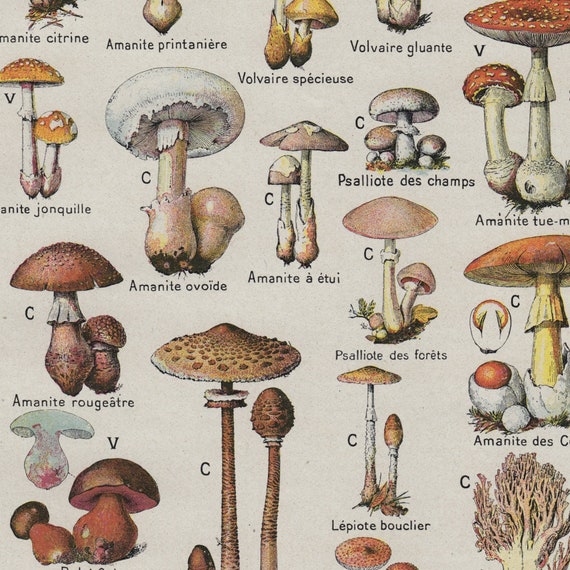The cropped image showcases a scientific illustration of various mushroom species against a grayish beige background. Each mushroom is depicted with its scientific name in black text below it. The mushrooms are generally shown in pairs, representing both their mature and immature forms. Many species are labeled with either a "C" or a "V," though the meaning of these labels is unclear. Notable mushrooms include one in the upper right with a red cap and white dots, paired with a smaller, all-white mushroom to its left. Yellow mushrooms feature prominently at the top, while brown and more abstract-looking mushrooms are towards the bottom. One notable mushroom in the bottom right resembles coral, and a tall, slender mushroom is visible near the bottom of the image. Some of the prominent species names mentioned include Amanite Ovoide and Saliote Deschamps. The image appears to be a section of a larger illustration, with some mushrooms and text cut off at the edges.